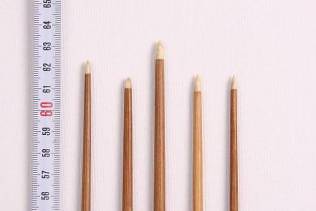The photograph is a close-up image featuring five writing or drawing tools, possibly paintbrushes or pencils, aligned vertically against a white background with slight shadows beneath them. A white ruler with black numbers is positioned vertically to the left of the tools, displaying a bold red "60" in the middle, with measurements ranging from 56 at the bottom to 65 at the top. Of the five tools, four have dark brown handles or bodies, while the second from the right has a lighter brown or pale red handle. Their tips are a light beige, blending with the color of the wood, and do not converge at the same vertical point. The leftmost tool is medium in height and the thinnest, the next one is shorter and thicker, the middle one is the tallest and thickest, the fourth is lighter in color and thinner, and the rightmost one is thin and about the same height as the fourth. The varying heights form a pattern: the leftmost reaches slightly higher, followed by a shorter one, then the tallest in the center, another shorter tool, and finally, the rightmost tool that matches the height of the second shortest.